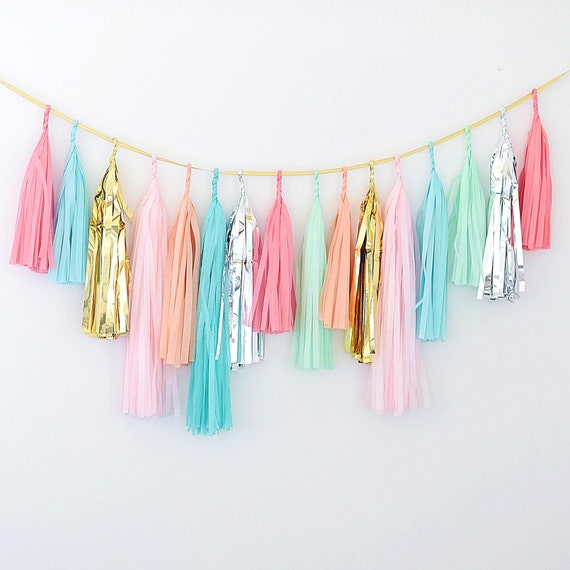In this image, a garland composed of various colored tassels — some made from thin plastic material and others from glimmering foil — hangs from a gold rope, fashioned to droop in a semi-U shape. The garland adorns a gray wall without any text in the frame. Beginning from the far left, the tassels display an array of soft, pale colors: a pink tassel resembling the fabric tendrils of a classic car washer or a cheerleader's pom-pom, followed by a light blue one. Moving right, a shiny gold foil tassel is slightly longer, leading to a delicate light pink tassel and then a shorter peach-colored tassel. Further along, there's another slightly longer blue tassel, a white one with a pattern, and a darker pink tassel. The garland continues with similar color patterns ending with another dark pink tassel positioned on the far right, matching the initial pink tassel on the left.